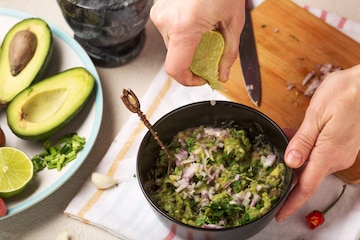This color photo provides a detailed, top-down view of a chef making guacamole. The scene centers on a black circular bowl containing mashed avocados garnished with purple onions, cilantro, and red chili peppers. The chef's left hand is holding the bowl steady, while the right hand squeezes a lime over the contents. To the right of the bowl, a round serving plate displays ripe avocado halves, one of which still contains its pit, alongside a half lime, a small clove of garlic, and diced scallions. An antique-looking spoon sticks out of the guacamole. A cutting board with a knife is positioned to the left side of the bowl. In the background, atop a kitchen towel, there's also a mortar and pestle at the top left corner of the photo. The overall scene is very clean and organized, highlighting the freshness and preparation of the ingredients.